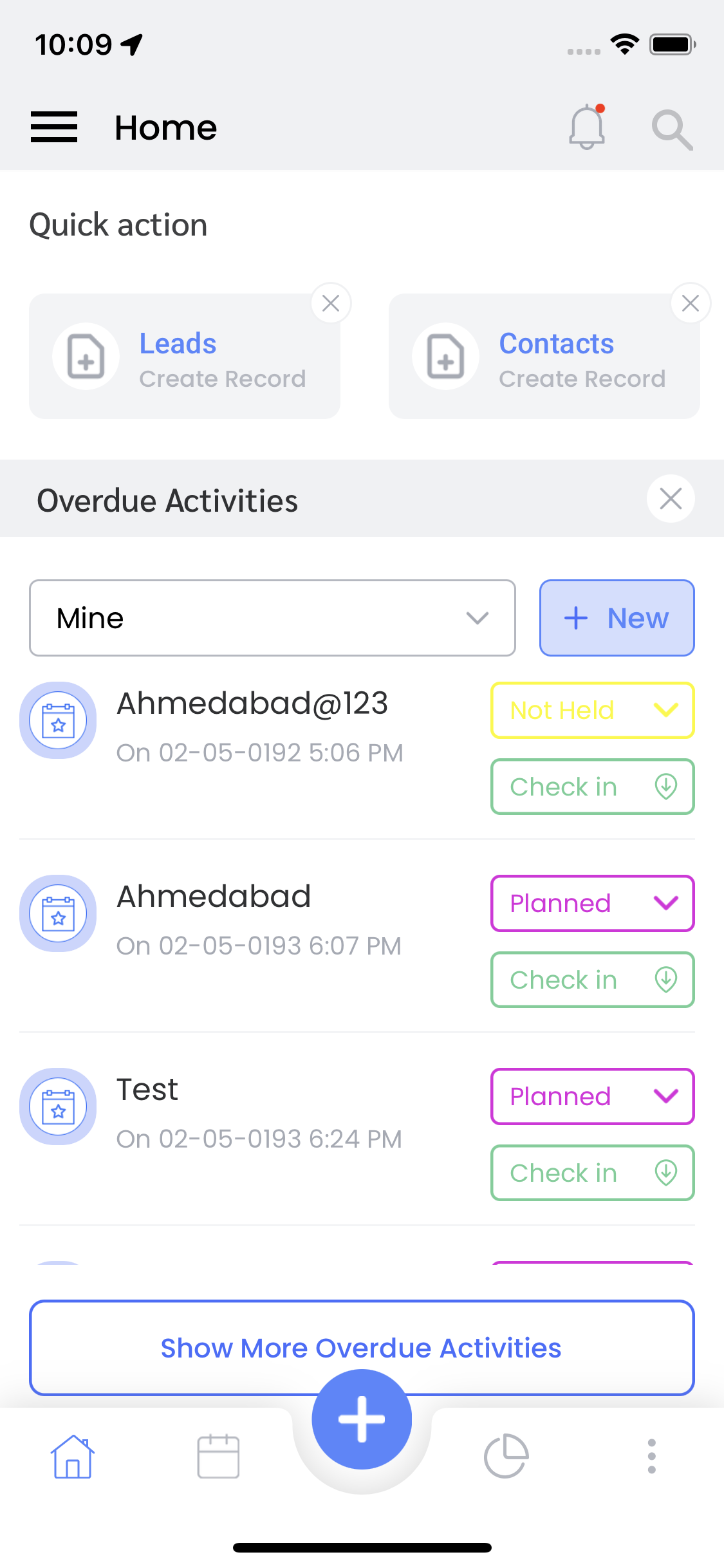The image is a screenshot of a mobile phone's interface displaying a home page with several interactive elements. At the top, there's a section labeled "Quick Action." Below this, two rectangular boxes labeled "Leads" and "Contacts" are visible, each containing a paper icon with a plus sign inside. The text "Leads" and "Contacts" is highlighted in blue.

Further down, there's a section titled "Overdue Activities" with a subheading "Mine." Within this section, there are clickable areas with a blue "Plus New" button.

The display includes a detailed list of activities with the following entries:
1. "Ahmedabad," timestamped "02-05-0192 at 5:06 PM," accompanied by a yellow box labeled "Not Held" and a green "Check In" button.
2. "Ahmed," featuring a purple box labeled "Planned" and a green "Check In" button.

Towards the bottom, there's another entry labeled "Test," maintaining similar interactive elements and color coding.